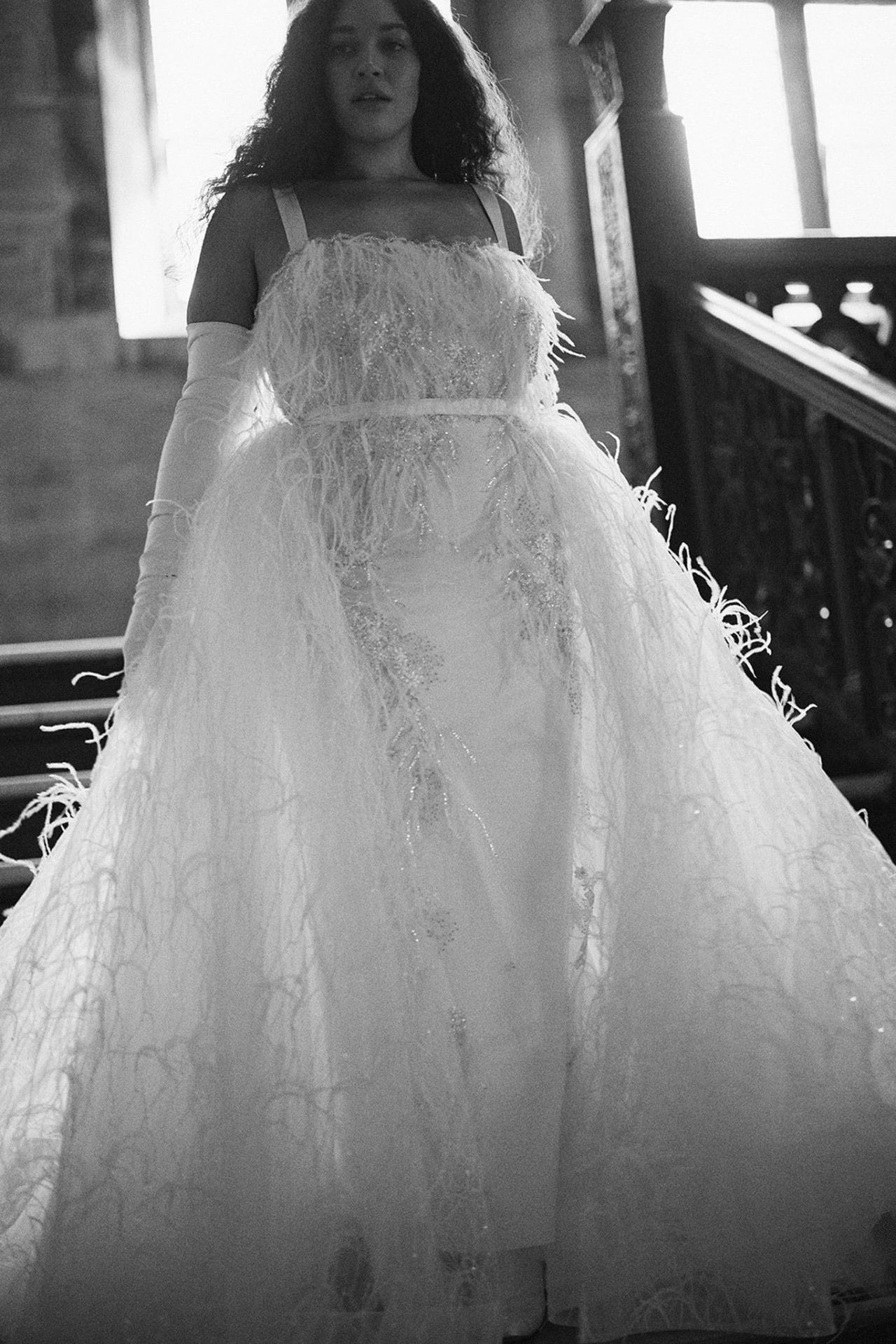In this black and white photograph, a woman in a striking bridal gown gracefully descends a staircase. The gown, sweeping and floor-length, is adorned with delicate, feathery, tassel-like structures, creating a flowing and voluminous effect. A prominent belt cinches the waist, adding definition to the ensemble. She is wearing long, fitted gloves that extend up to her upper arms, complementing the ethereal nature of her attire. The woman has long, dark, slightly curly hair cascading over her shoulders, and she gazes off to the left, a serene expression on her face.

The setting suggests a blend of old-world charm and industrial simplicity, with stone or cement walls visible in the background. A faint, blurred view to the right shows more of the setting, potentially resembling a warehouse. The staircase she descends has dark grey railings, and there is a window directly behind her, casting a soft, luminous light around her figure. Another window is situated at the top right of the image, enhancing the photograph's atmospheric lighting. The overall theme underscores the significance of the moment, capturing the beauty and grace of the bride on her wedding day.